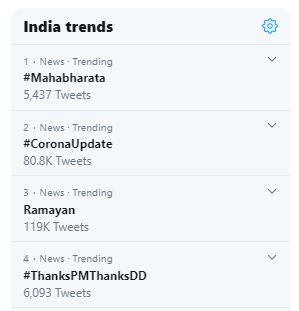The screenshot showcases the trending topics in India. In the upper right corner, a blue settings icon is visible. To the left, bold black text reads "India Trends." The first trend is "News Trending" with the hashtag #Mahabharata, accompanied by 5,437 tweets and a pull-down arrow to the right. The second trend, "News Trending," features the hashtag #CoronaUpdate, with 80,800 tweets and a corresponding pull-down arrow. The third spot is occupied by "News Trending" followed by the bold text "Ramayan," which has garnered 119,000 tweets, also with a pull-down arrow. Lastly, in the fourth position under "News Trending" in bold black text, the hashtag #ThanksPMThanksDD is listed, having accumulated 6,093 tweets.